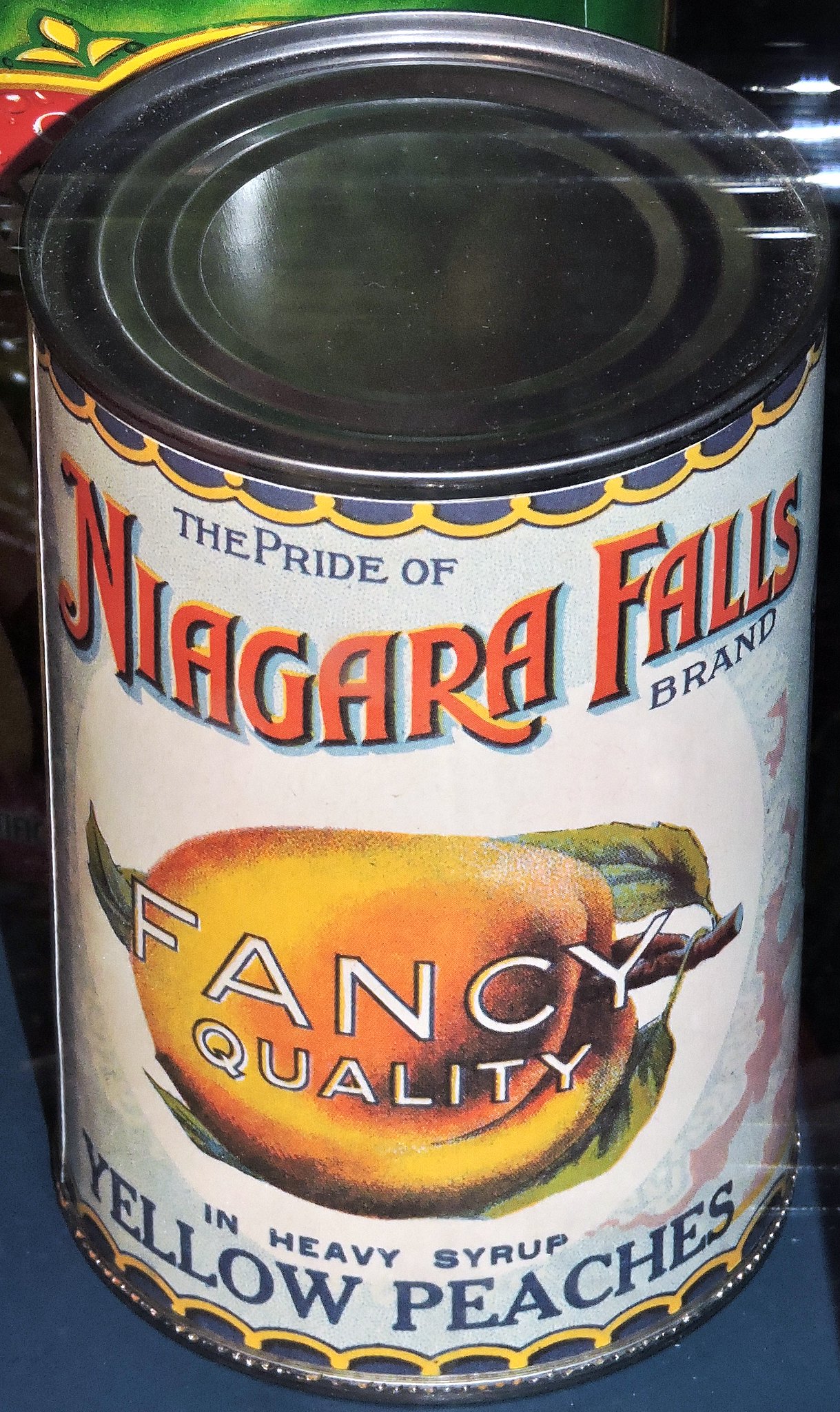A meticulously designed can of peaches is adorned with an intricate print that wraps around the entire surface. The primary background color is white, with the top and bottom sections featuring a vibrant blue and yellow embroidered pattern resembling half-petals encircling the can. The label prominently reads "The Pride of Niagara Falls Brand" and "Fancy Quality" in smaller blue print, as well as "In Heavy Syrup" also in smaller blue print. The standout text, "Yellow Peaches," appears in bold blue letters, while "Niagara Falls" is prominently showcased in bold red lettering. At the center of the label is an illustration of golden-orange peaches clinging to a branch, accompanied by two lush green leaves partially overlapping the fruit. Hovering above this central image, the words "Fancy Quality" are emblazoned in bold white letters, completing the visually appealing and descriptive package design.